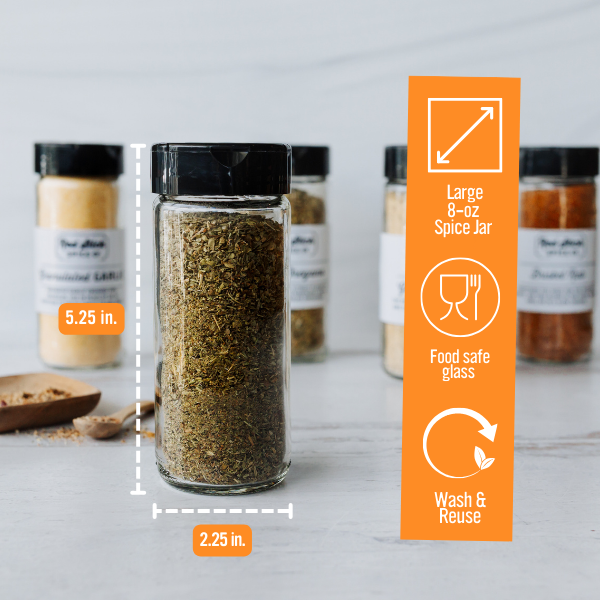This detailed photographic image showcases a set of six clear glass spice jars with black lids, displayed indoors against a white background that resembles quartz or marble, likely in a kitchen setting. Five of the jars, sitting in the back, are out of focus and filled with various spices, distinguishable by their different colors: whitish-yellow, dark green, whitish, and reddish-brown. They all have small white labels identifying their contents.

In the forefront, a single jar is in sharp focus, containing finely crushed green spices, possibly dill or parsley. This jar has detailed measurements highlighted by dashed lines indicating its dimensions: 5.25 inches high and 2.25 inches wide. To the left of the jar, an orange bubble reiterates the 5.25-inch height. 

To the right of the jar, an orange rectangle presents additional information, featuring a symbol of a square with diagonal arrows and the text "Large 8-ounce spice jar." Below this, symbols and text convey that the jar is made from food-safe glass and can be washed and reused, represented by an icon of a fork and glass within a circle that transitions to a counterclockwise arrow ending in a leaf. A small squarish spice tray with a spoon and spilled spices is also part of the scene, enhancing the kitchen ambiance depicted.